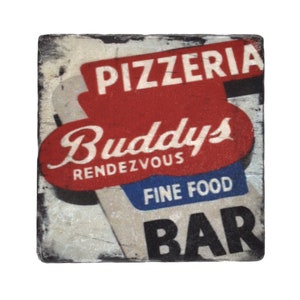This is a small, vintage square image advertising "Buddy's Rendezvous Pizzeria, Fine Food & Bar." The top section features the word "Pizzeria" in bold, white, all-capital letters on a red background, giving a worn and aged aesthetic. Below, "Buddy's Rendezvous" appears with a capital "B" followed by lowercase letters, with "RENDZVOUS" in smaller, all-capital white letters. The phrase "Fine Food" is displayed in white, all-capitals on a blue background beneath this, and finally, the word "B.A.R." stands out in large black letters. The image, with its faded colors and slightly altered edges, exudes a nostalgic, rustic charm, typical of old sign styles, possibly hinting at a cozy eatery serving pizza, meals, and alcoholic beverages.